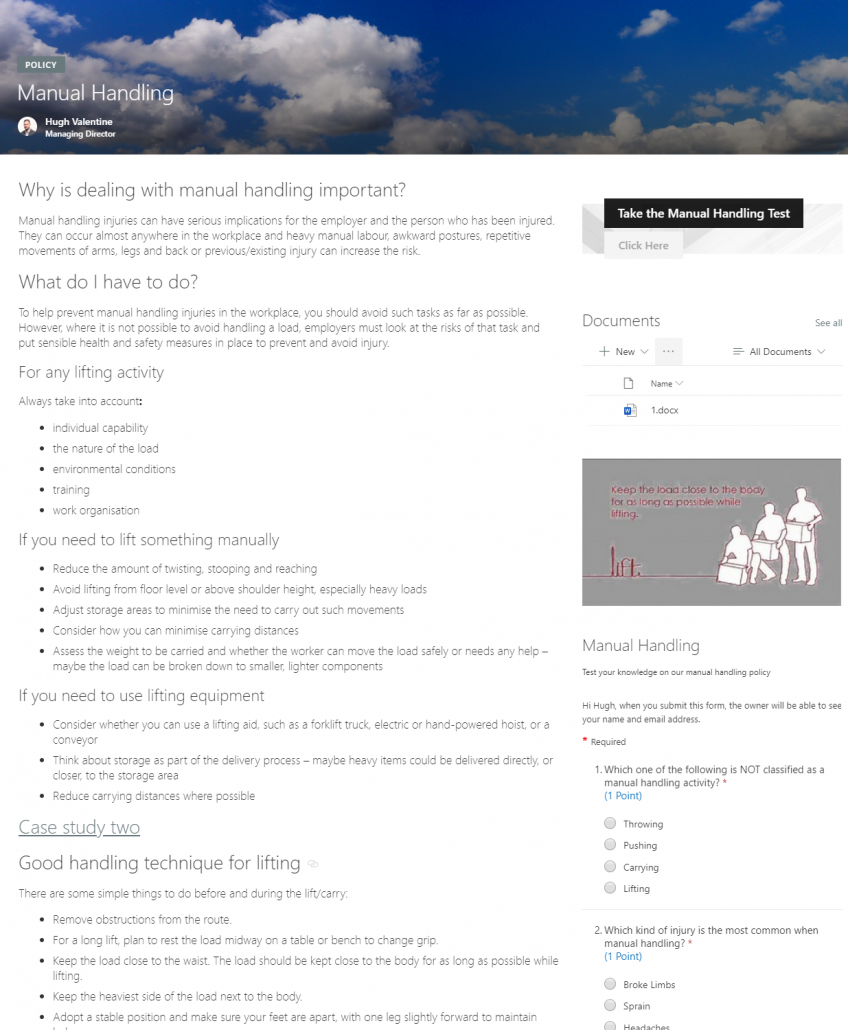This image features a predominantly white background filled with a variety of informative text. At the top, stretching across the screen, there is a long, narrow image depicting a blue sky adorned with white clouds. Towards the left of this image, the word "Policy" is prominently displayed, followed by the phrase "Manual Handling."

Below this, on the left side, there is a small circular photograph featuring a dark-haired white man. On the right side of this photograph, the text reads "Hugh Valentine, Managing Director." 

Beneath the photograph, the content is divided into several sections with bold headers. The first header asks, "Why is dealing with manual handling important?" This section elucidates the significance of proper manual handling practices. The next header poses the question, "What do I have to do?" Underneath, a paragraph provides detailed instructions on manual lifting.

One noteworthy piece of advice is: "For any lifting activity, always take into account individual capability, the nature of the load, environmental conditions, training, work organization." The article stresses the importance of minimizing twisting, stooping, and reaching while lifting. It specifically advises against lifting from floor level or above shoulder height, particularly when dealing with heavy loads.

Further down, the text recommends considering lifting aids such as forklift trucks, electric or hand-powered hoists, or conveyors when equipment is necessary. Adjacent to this information, a small gray box contains an illustration demonstrating the correct lifting technique. This visual guide shows an individual bending their knees and lifting with their legs while maintaining a straight back to prevent injury.